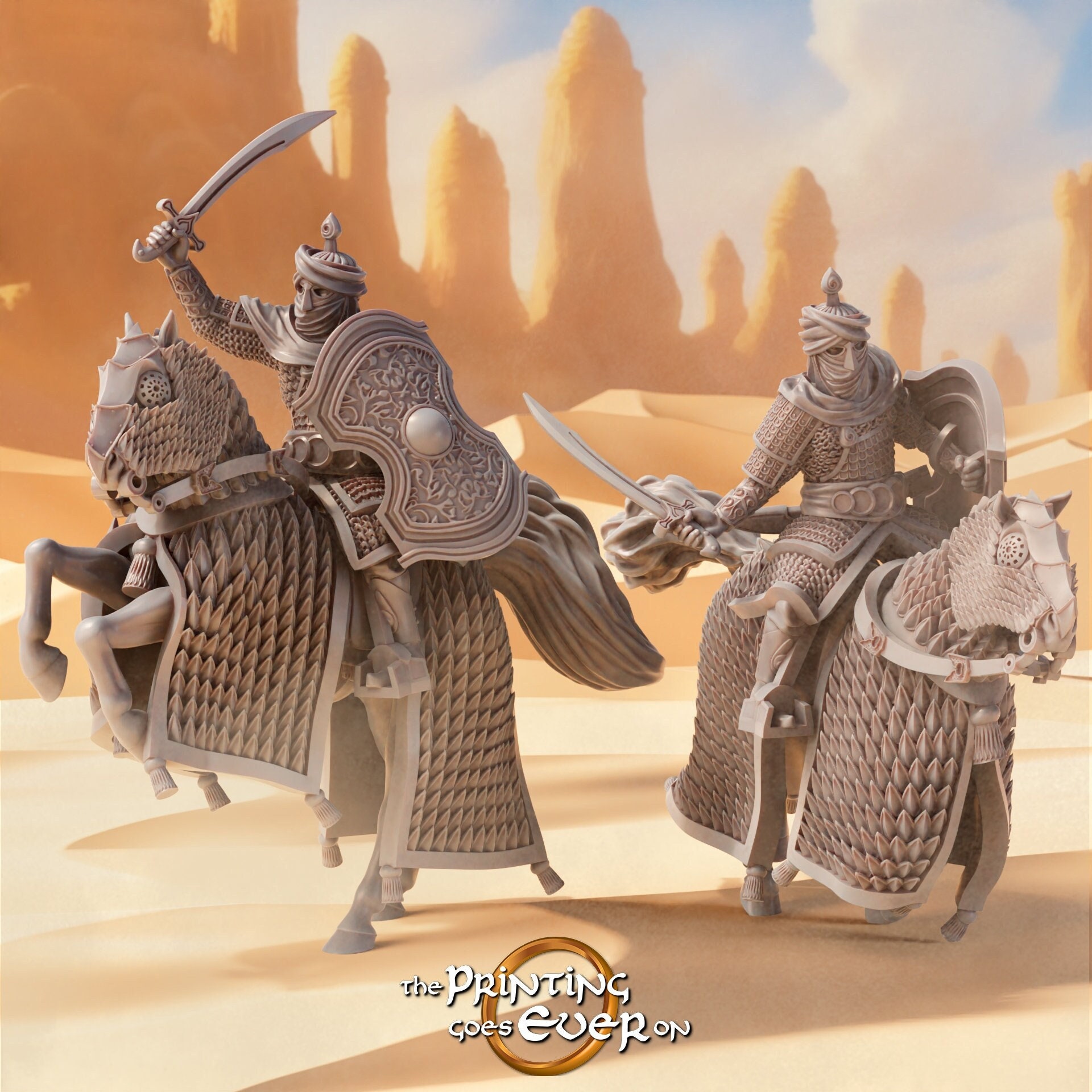The image is a detailed 3D rendering, possibly a poster or cover for a video game, movie, or animation titled "The Printing Goes Ever On." The title text appears at the bottom center in white font with a golden ring as a backdrop, reminiscent of the Lord of the Rings logo. The scene depicts two knights on horseback, both entirely in shades of light gray with no other color information. These warriors are fully armored, including their horses, and they wield swords and shields. Their faces are obscured by face scarves and either helmets or turbans. The backdrop is a vast desert-like terrain with a blue sky and white clouds, featuring a sandy castle or tall mounds of sand in the background, creating a cohesive and intricate medieval desert scene.